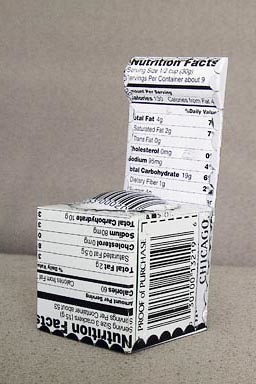The image presents a meticulously detailed view of a black and white square-shaped box placed against a monochromatic gray backdrop. Both the wall and the table on which the box rests share this gray tone, creating a subtle yet uniform background. 

Attached to the rear of the box, a tag extends upward, prominently displaying nutritional information. This tag details specifics like total fat, cholesterol, sodium, and total carbohydrates. On top of the box, there's a visible barcode, adding a layer of practical detail.

The front of the box prominently features a label that reiterates the nutritional facts, again listing calories, total fat, cholesterol, sodium, and total carbohydrates. Meanwhile, the box's right-hand side displays another barcode, labeled "proof of purchase," with the word "Chicago" inscribed just below it. The barcode is numbered 5-0-1-3-2-1-9, offering a precise identifier to this otherwise minimalist packaging.